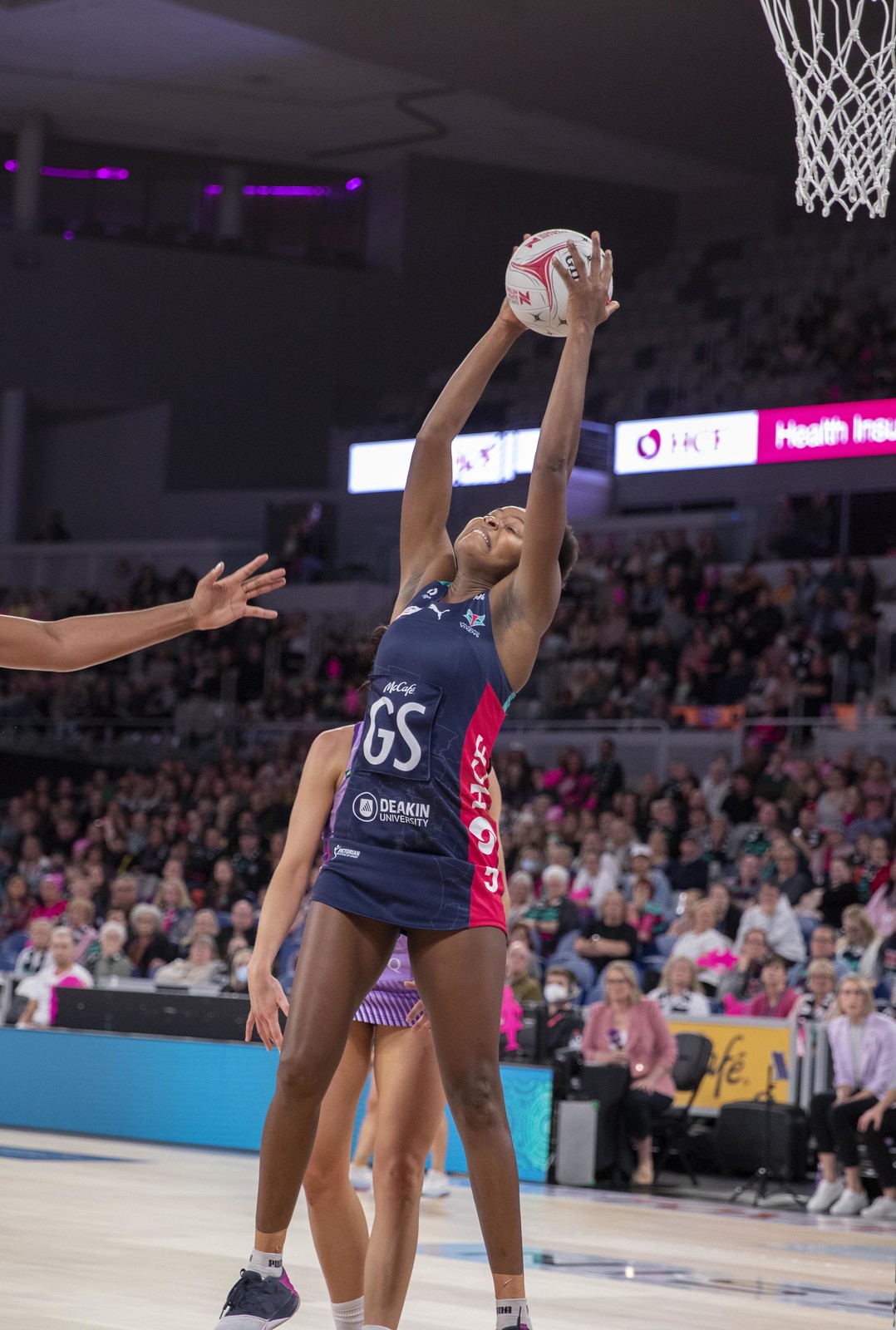In this vibrant full-color photograph taken at an indoor women's basketball game, you can see a dynamic moment captured on the wooden court. The central figure is a young African American woman, mid-jump, clad in a distinctive blue and red uniform with prominent white letters "GS" on the front. She holds the basketball high above her head, possibly indicating she has just grabbed a rebound or is preparing to make a play. Behind her stands another player in a purple uniform, suggesting an opponent trying to challenge or guard her. To the left edge of the frame, a left arm reaches toward the central player, intensifying the action.

The background is bustling with activity; the stands are packed with spectators, their identities blurred, filling tiered bleachers that ascend at least two levels. At the top tier, there is a concourse area, partially lit and holding what appear to be skyboxes, with one illuminated by purple lights. Brightly lit advertising signs for sponsors cast a glow over sections of the crowd, contributing to the lively atmosphere. In the upper right corner of the photo, part of the basketball hoop and net can be seen, framing the action and setting the stage for this tense moment in the game.